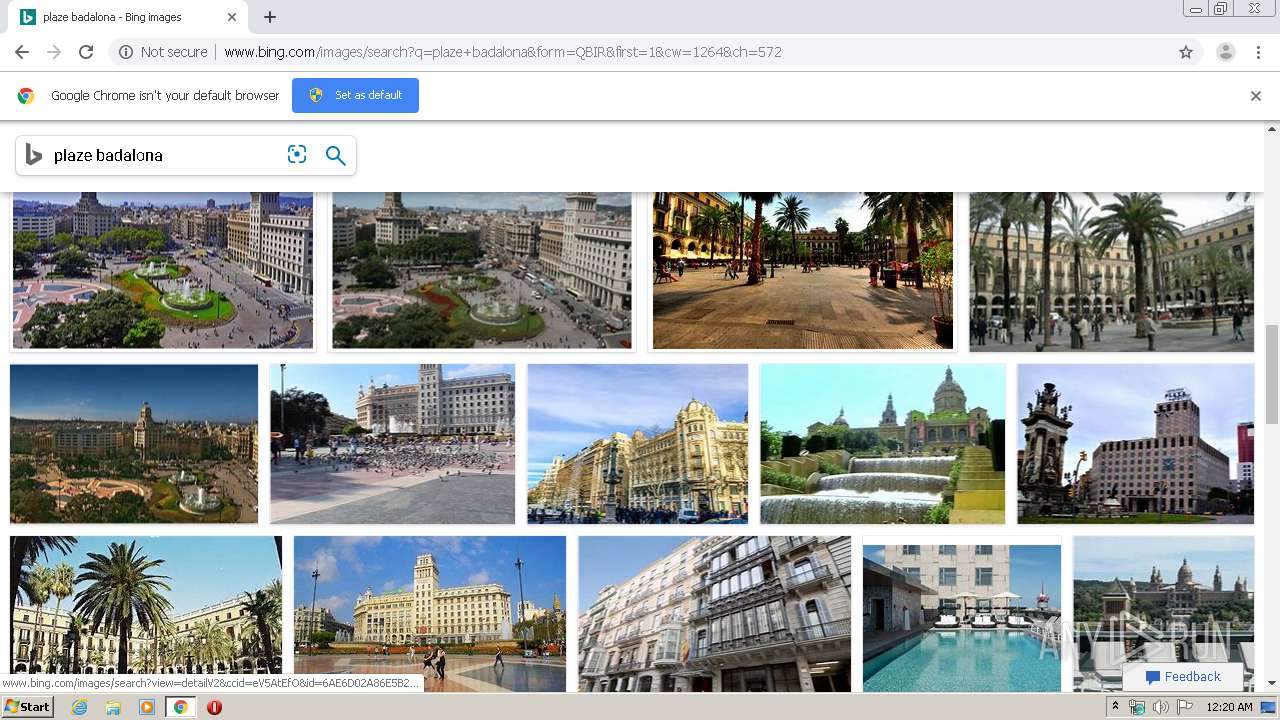Detailed Caption:
The screenshot features a web browser window open on a desktop, likely emulated to resemble a vintage Windows 95 environment. At the very top of the screen, there is a white bar on the left containing an open tab with illegible black text due to its small size. Adjacent to this bar is a black plus sign followed by a gray bar stretching to the right. The upper right corner presents the typical closeout buttons for minimizing and closing the window.

Below the top bars, a browser navigation bar is visible. On the left side, there are black and gray arrows for navigating back and forth, followed by a circular refresh icon. The address bar displays "bing.com," indicating the search engine in use. To the right of the address bar, icons for bookmarking (a star), user account (a person), and additional settings (three vertical dots) are lined up.

Underneath this navigation bar, a notification prompts to set "Google" as the default browser, featuring Google and Chrome logos and an option labeled "Set Now." The main content of the browser window shows search results for "Plaza Barcelona," displaying numerous high-definition images of the downtown area of Barcelona. These images include several perspectives of a spacious, verdant plaza, a bustling public square adorned with palm trees, and impressive architectural landmarks that could be municipal buildings, such as a city hall.

At the very bottom of the screen, a gray taskbar with the nostalgic Windows 95 Start logo and icons is present, hinting at the emulation or retro customization of the operating system being used to run the modern Chrome browser.